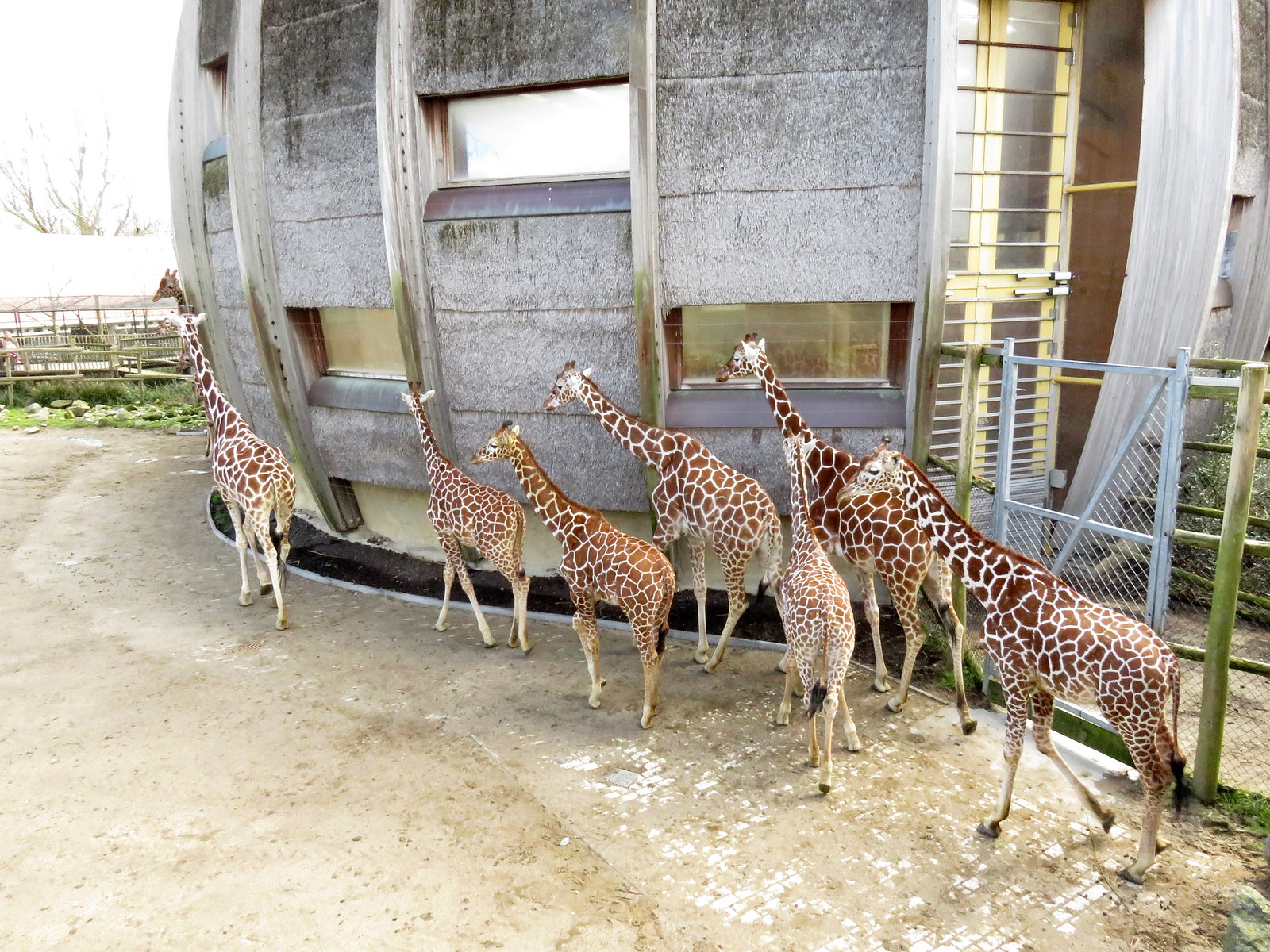This image captures a group of seven to eight young giraffes walking along a mixed cobblestone and dirt path. They are closely hugging a large concrete building with sporadically placed windows that resemble a caged enclosure, most likely where the giraffes sleep at night. The building is constructed with concrete blocks and has steel reinforcements running between the windows, enhancing its sturdiness. The giraffes, varying in shades of brown with distinct white markings, are led by an adult giraffe and appear to be making their way towards a feeding area that is marked by patches of grass and food visible on the ground. To their right, a steel grated fence encloses the path, adding to the sense of confinement within the area. The scene captures the giraffes walking purposefully towards the left, with a hint of a garden visible behind them.